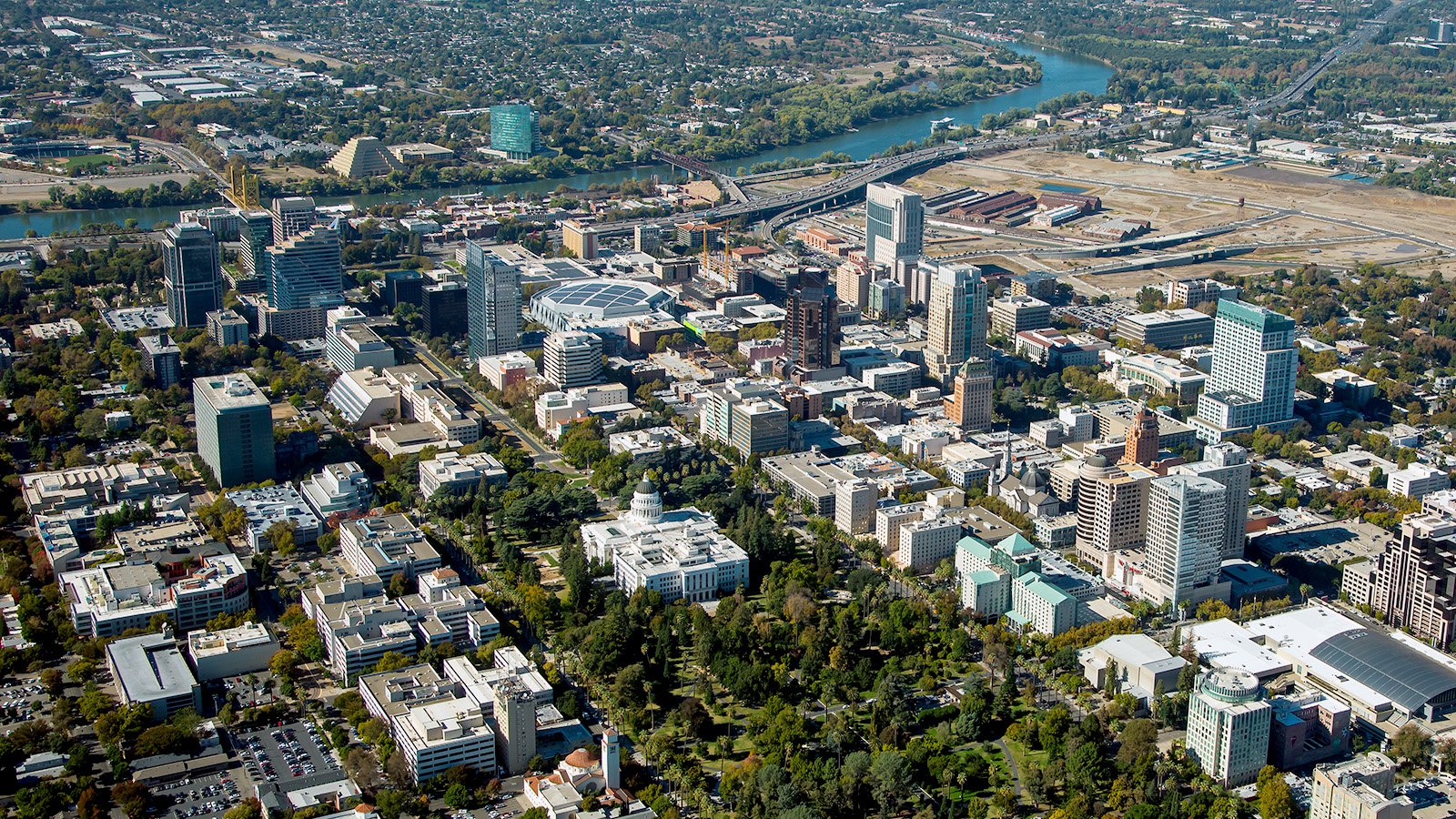This aerial photo captures a sprawling cityscape dotted with greenery and park areas stretching into the distance. The image prominently features a meandering river that winds from the top left across to the right before curving upward and vanishing out of sight. A striking yellow bridge spans the river, linking the urban landscape on either side. Near the center, several tall skyscrapers rise up, including a distinctive circular building almost mid-center. In the backdrop, a notable pyramid-shaped building catches the eye, with a large blue-facade structure to its right. The upper right quadrant is densely packed with residences, while the left side reveals a construction zone characterized by lots of dirt and elongated, red metal sheds. Highways with active traffic run parallel to the river, contributing to the city’s dynamic energy. Amidst this architectural grid, patches of trees and potential city parks soften the urban rigidity, creating a harmonious blend between nature and city life.